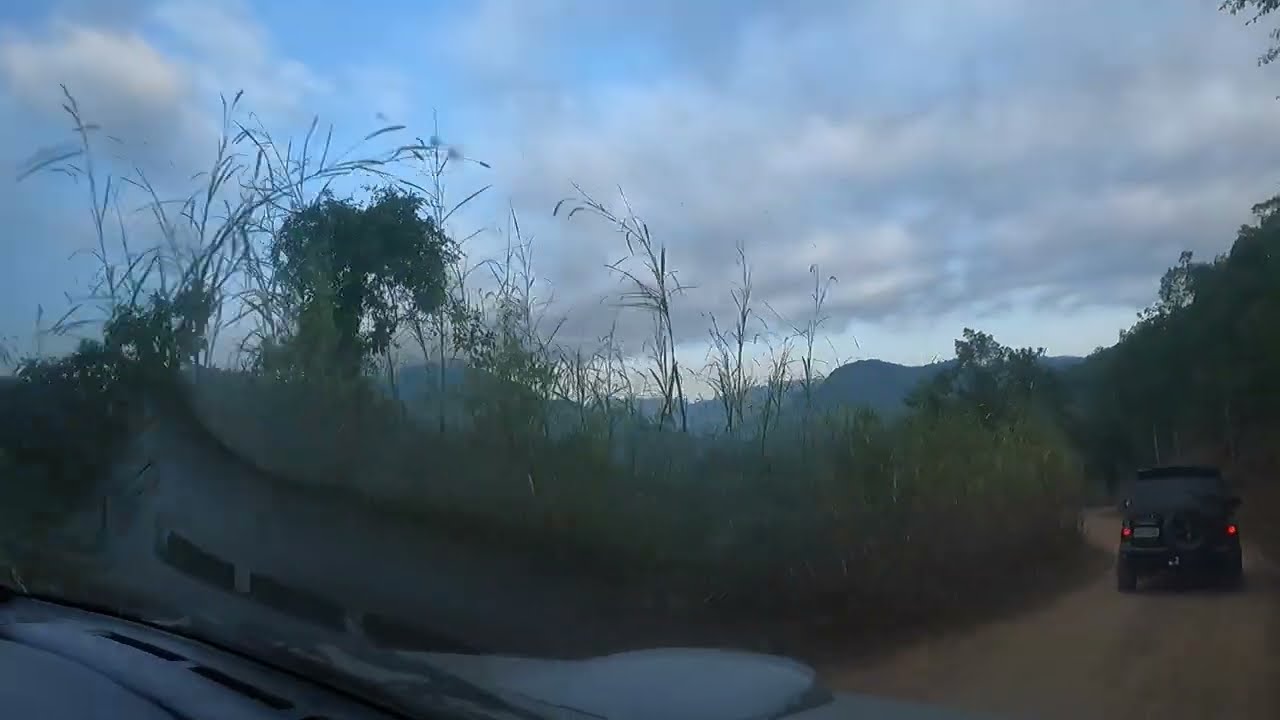The photograph, taken from inside a vehicle and through its windshield, captures a curvy dirt road located in the bottom right corner. This narrow, winding road snakes through a landscape thick with overgrown grasses and tall weeds on the left side, while small trees and a slightly elevated patch of land reside on the right. Dominating the right side of the road is a black SUV or Jeep, characterized by its conspicuous rear-mounted tire and illuminated taillights, suggesting it is in motion. In the far distance, rolling hills or a mountain emerge against a partly cloudy, blue sky that becomes increasingly gray and cloudy towards the right. Additionally, the lower left corner of the image shows the vehicle’s dashboard and vents, with their reflection visible in the windshield.